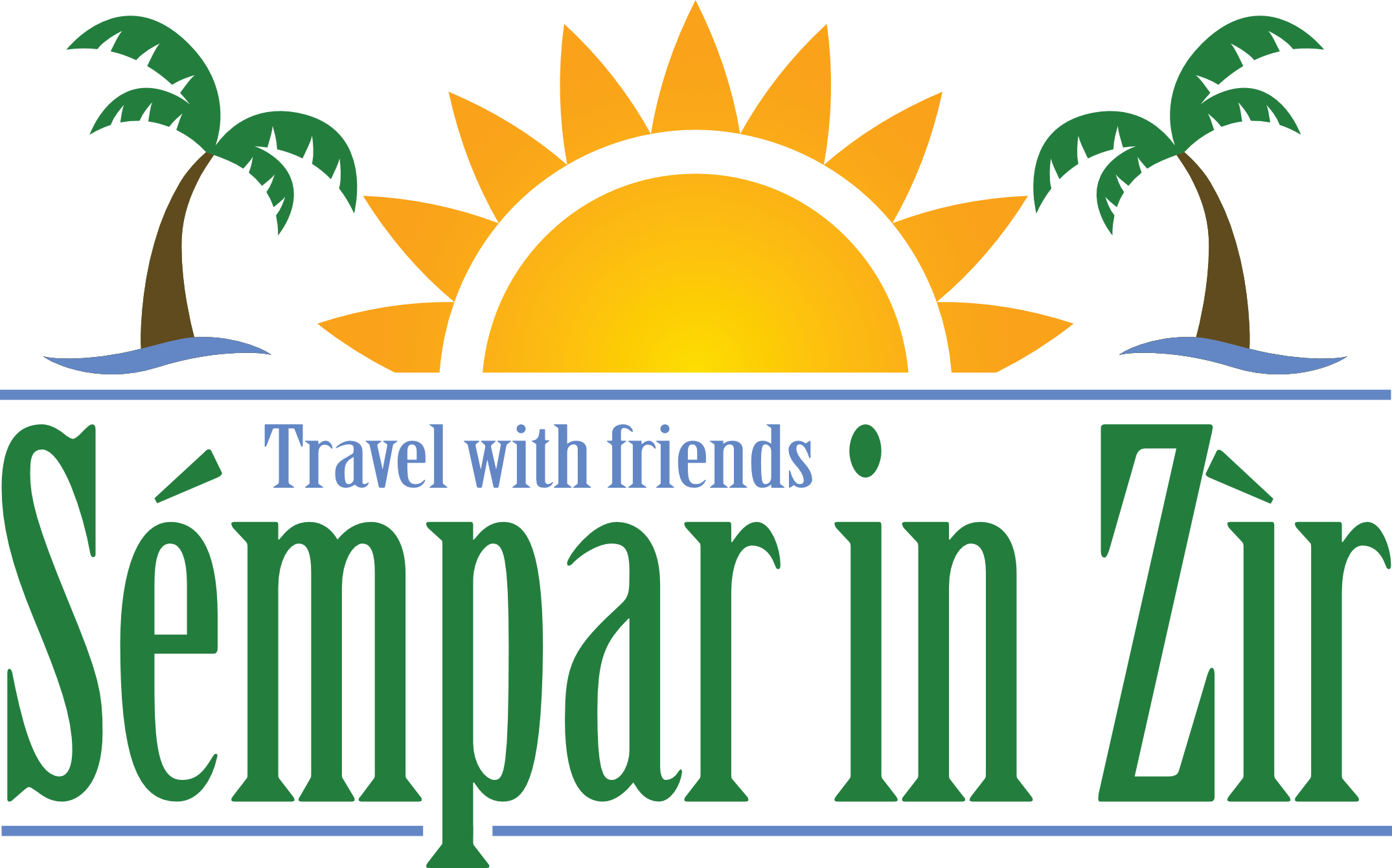The image depicts a company logo on a solid white background, featuring a tropical-themed graphic. Centrally aligned, the upper portion includes a stylized, half-circle yellow sun with orange rays, bordered by a white outline. Flanking the sun on both the upper left and right corners are two palm trees, each with a brown trunk and green leaves arching inward towards the sun. Beneath the sun is a horizontal blue line, mirrored by another at the bottom of the image, enclosing the text. The large green font reads "Sempar Inzir," with the smaller blue text "travel with friends" positioned above the word "Sempar." The overall style is cartoony, suggestive of a travel agency branding, and uses a palette of white, green, brown, blue, yellow, and orange.